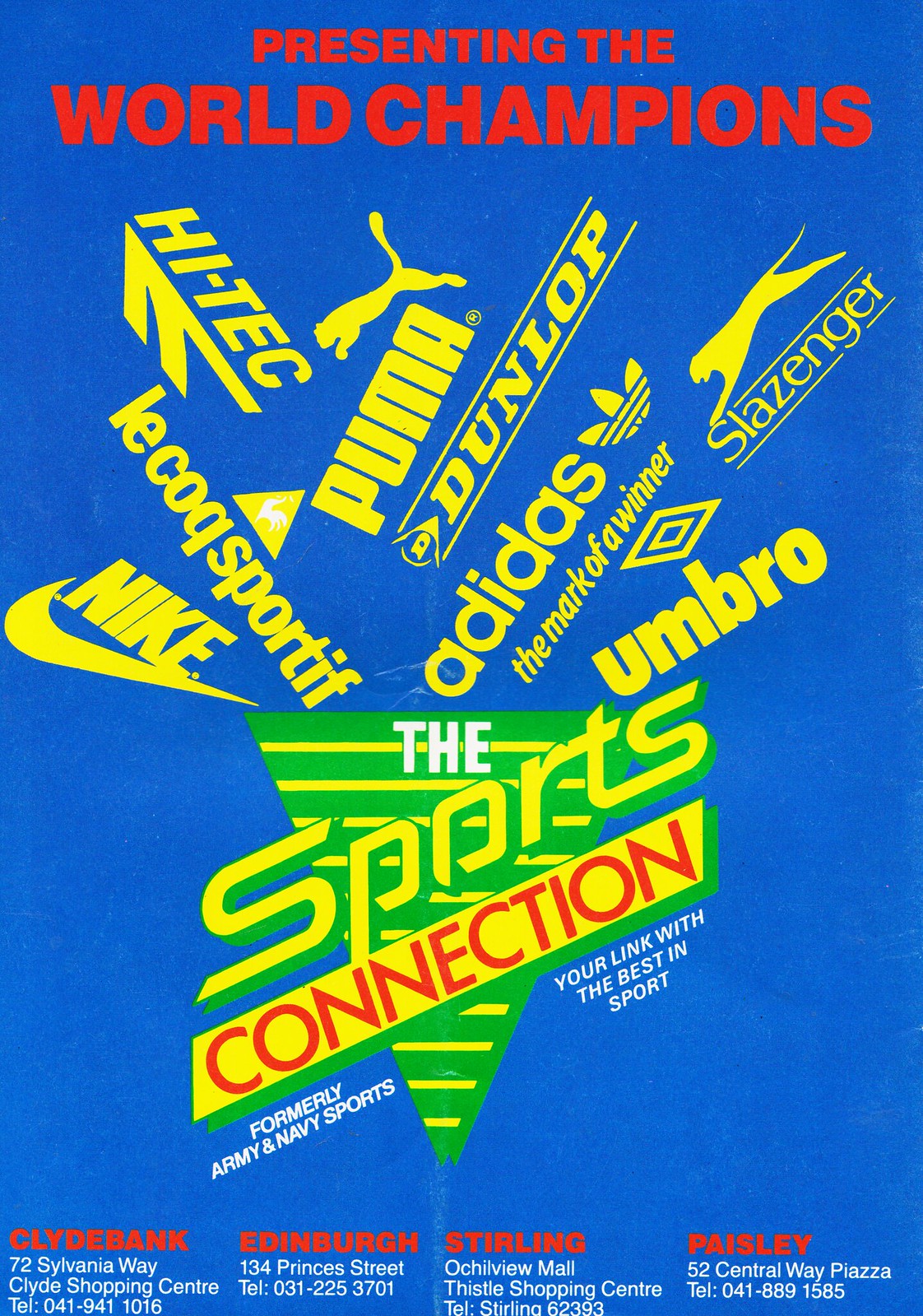This image features an advertisement poster with a blue background and an upside-down yellow and green triangle prominently displaying the text "Sports Connection" in red. The poster, formerly associated with Army and Navy Sports, bears the tagline "You're linked with the best in sports." Various sports brands, including Nike, Hi-Tech, Le Coq Sportif, Puma, Dunlop, Adidas (the Mark of a Winner), Slazenger, and Umbro, are showcased within the triangle. The lower section provides contact details for several store locations: ClydeBank at 72 Sylvania Way, Clyde Shopping Center (Tel: 041-941-1016); Edinburgh at 134 Princes Street (Tel: 031-225-3701); Stirling at Oakview Mall, Thistle Shopping Center (Tel: Stirling 62393); and Paisley at 52 Central Way, Piazza (Tel: 041-889-1585).